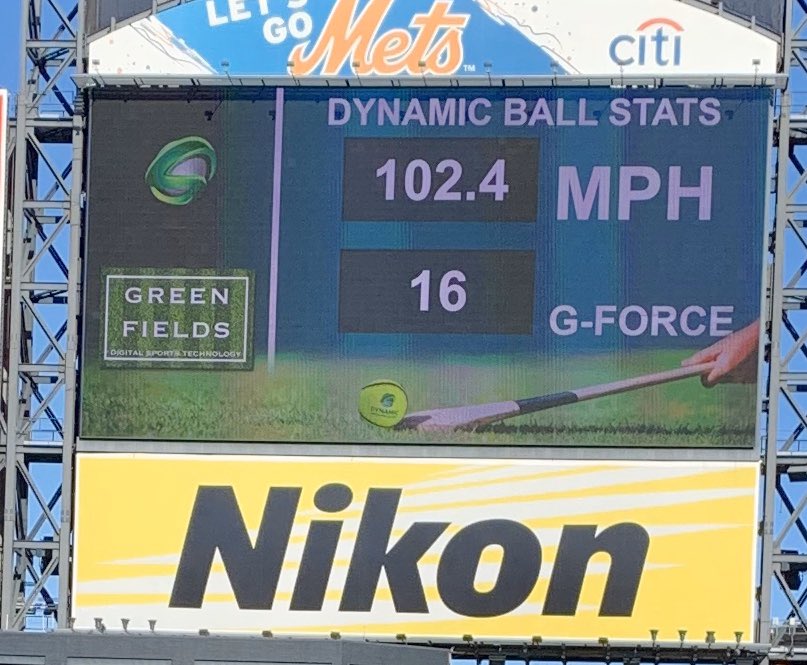The photograph is a full-color image, likely taken outdoors using natural light, and depicts an informational board at a sporting event, possibly a baseball game. The square image, without a definitive border or background, showcases a blue sky and metallic girders along the left and right sides that support the sign. At the top, the sign prominently reads "Let's Go Mets," indicating it is associated with the New York Mets and suggests a baseball context. This is further emphasized by the sponsorship by Citibank, hinting at Citibank Field. The central portion of the sign is digital, displaying the text "Dynamic Ball Stats" with detailed statistics: "102.4 miles per hour" and "16 G-Force." The image includes an illustration of a bat hitting a ball that resembles a yellow tennis ball. Additional sponsors mentioned include "Greenfield's Digital Sports Technology" and "Nikon," with Nikon's logo positioned at the bottom of the sign. Overall, the image appears to be a digital display for batted ball statistics at a Mets game.